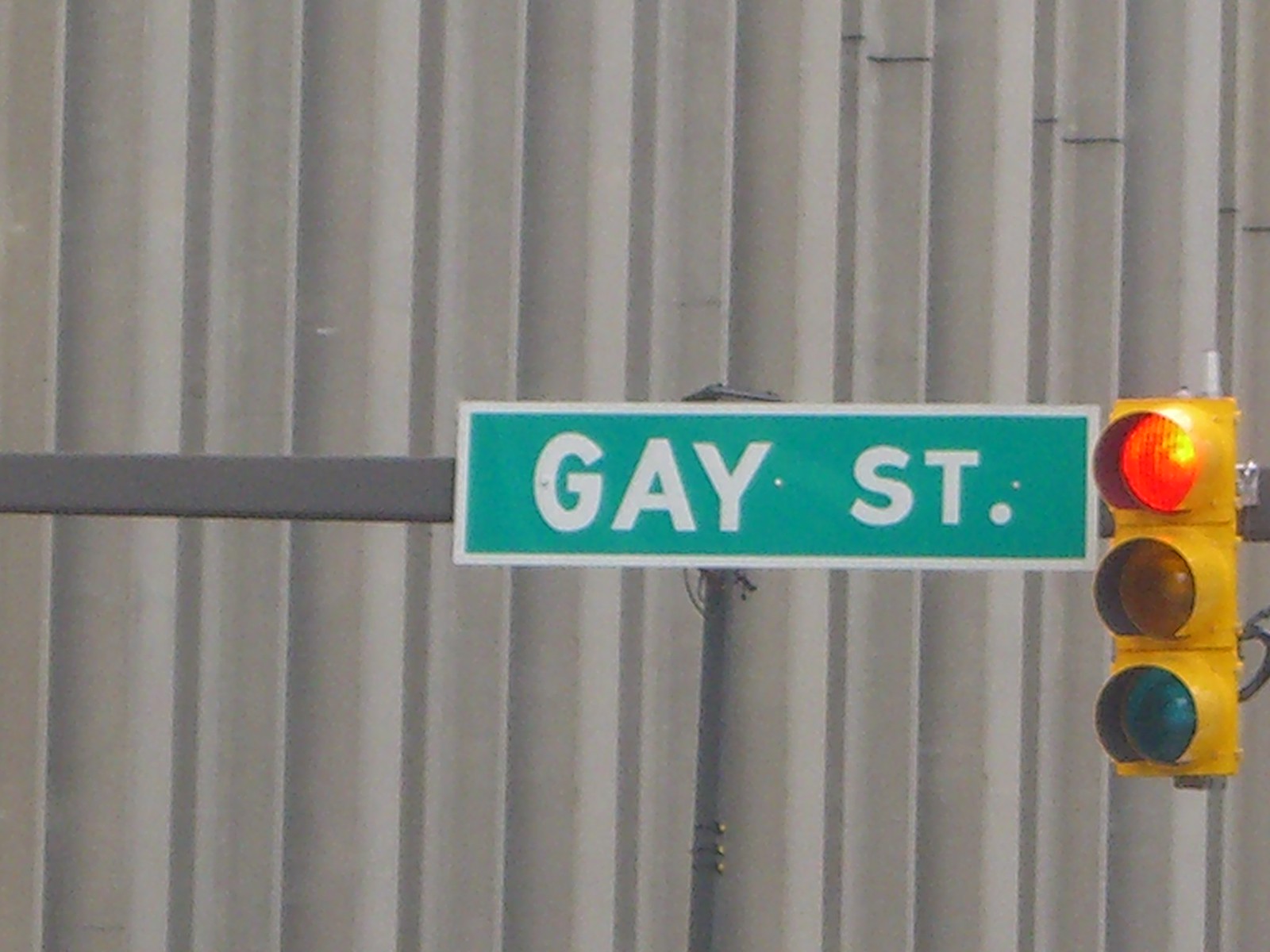The photograph captures a street scene dominated by a tall, greyish-brown building or wall with vertical ridges in the background. A prominent street sign with a green rectangular design and white text reads "Gay ST." and is held up by a silver metal bar extending horizontally from the left side of the image. Adjacent to the sign on the right is a bright yellow traffic light, currently illuminated in red at the top, signaling a stop. The well-defined elements create a vivid urban tableau.